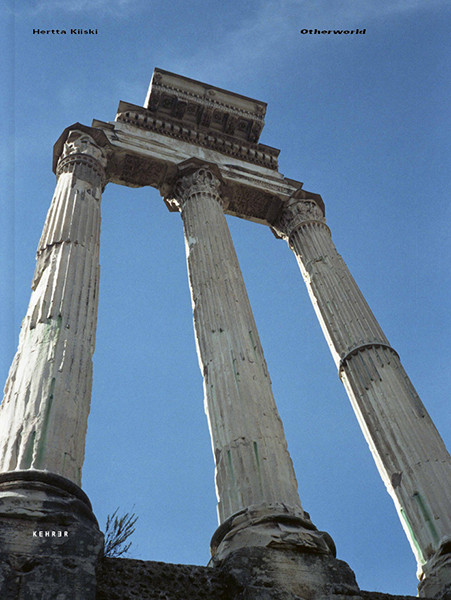The photograph depicts three towering, greyish-white Corinthian stone pillars, remnants of an ancient structure, possibly from ancient Greek times. Each column is heavily weathered, showing significant damage with chipped edges, cracked surfaces, and missing chunks. Atop the pillars rests a partial ornate stone wall, featuring intricate details and a small segment of ceiling that precariously hangs over the structure. A bit of green foliage is visible between the first and second columns, adding a touch of nature to the scene. The background showcases a clear blue sky with just a hint of white haze near the top, enhancing the prominence of the ancient ruins. The image appears to be of low quality and might be a book cover, as there are titles and names such as "Herakleski," "Otherworld," and "Cahir" displayed in the corners.